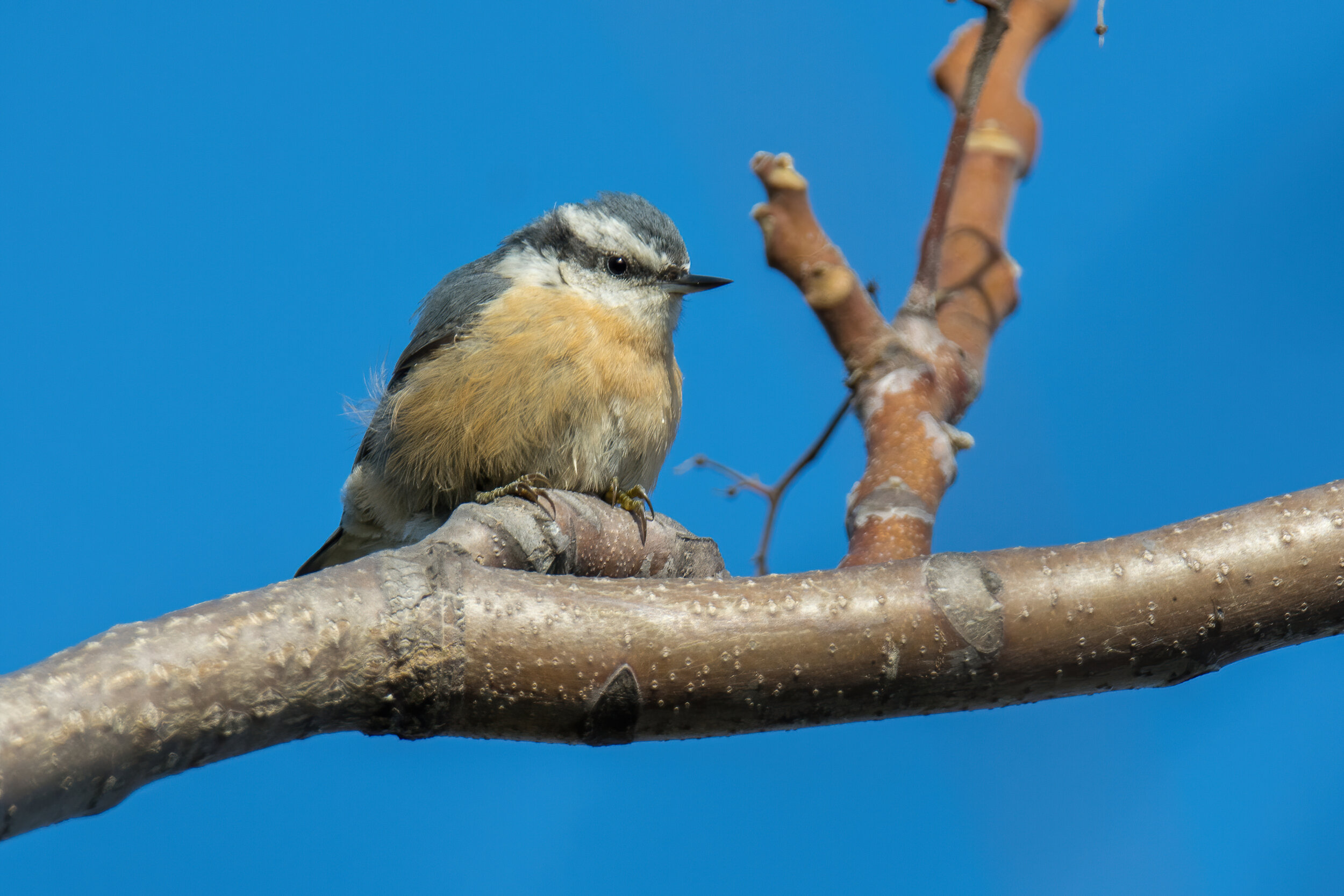The image is a horizontal rectangular photograph capturing a small bird perched on a branch. The bird features a distinctive black beak and eye, complemented by a striking black stripe that extends from the beak, passes through the eye, and continues to the back of the head. Flanking this black stripe are patches of white feathers. Another black stripe runs over the top of the bird's head. The bird's chest and underside are adorned with beige-brown feathers, while its upper wings display a blackish-gray hue. The bird's two feet are firmly gripping a branch that extends away from the viewer. Another branch, brown in color, runs horizontally from left to right behind the bird, and a third branch ascends vertically on the right side of the image. The background is filled with a beautiful, blurred scenery that adds a sense of depth and focus to the bird.